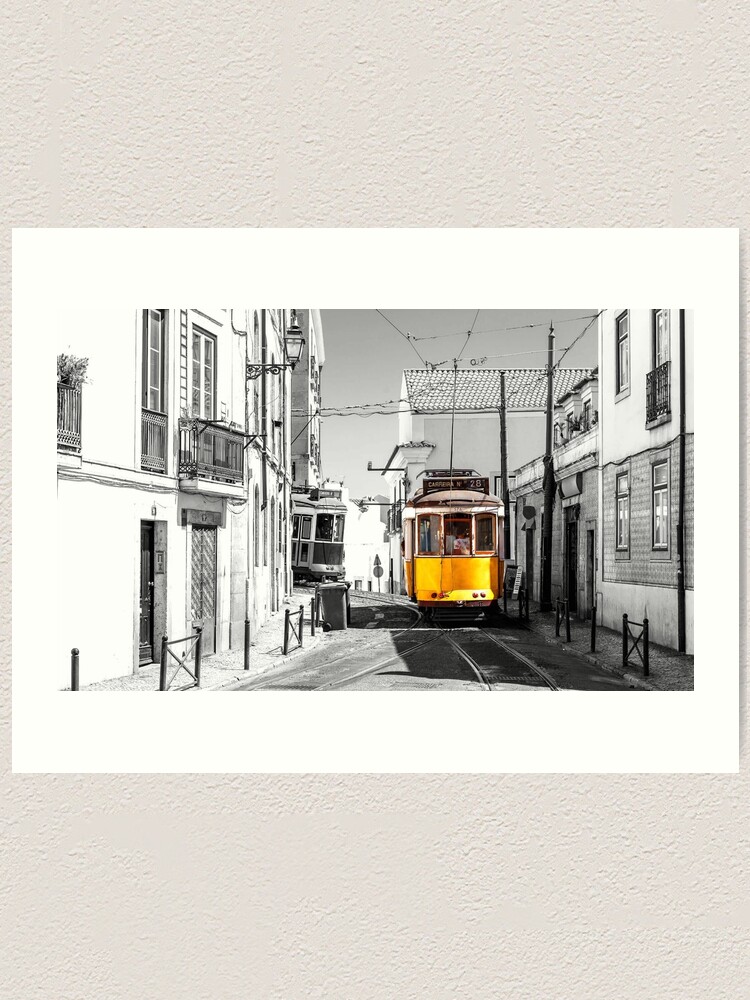The image is a black and white photograph, selectively colorized by what appears to be hand-tinting with watercolors. It features a narrow street, flanked by older buildings that are adorned with iron balconies on the second story. These buildings continue into the distance on both sides of the street. A bright orange-yellow cable car, accented with brown, dominates the scene as it travels up the street. Visible power lines stretch overhead, and the tracks for the cable car run along the road. Plant boxes are perched on some of the balconies, and a stop sign can be spotted in the background. The photograph, in landscape orientation, is printed on high-quality archival paper with a broad white border. This is presented against a textured white background, adding an additional layer of depth to the overall composition.